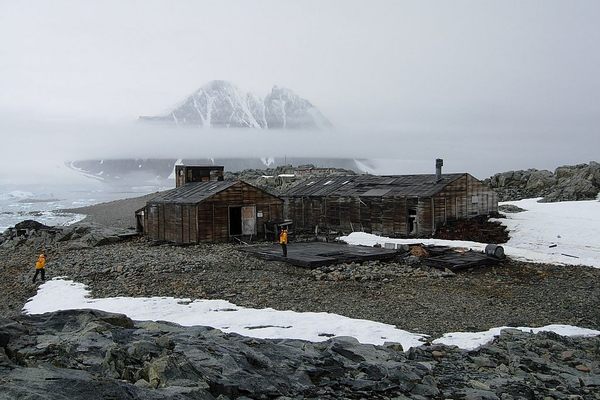The image depicts a cold, bleak scene dominated by a large, weather-beaten log cabin and an additional dilapidated cabin beside it. The cabins appear worn and stained, potentially due to the harsh weather conditions, resembling an outpost in an isolated, rocky area. The sky is an unbroken expanse of gray, heavy with moisture, adding to the overall feeling of cold. In the background, faintly visible through the mist, are mountains with a blend of white snow and dark gray rock, contributing to the desolate atmosphere. The ground is mostly blackish-gray gravel with sporadic patches of snow, and there is no vegetation in sight. In the foreground, two people in yellow or orange jackets with black trousers are present; one is walking towards the building while the other stands nearby, suggesting they might be workers, possibly involved in scientific research. Additionally, a cylindrical drum lies on its side, and the sea meeting the rocky shore can be glimpsed to the left, enhancing the sense of a remote, inhospitable location, possibly somewhere in Scandinavia or even Antarctica.